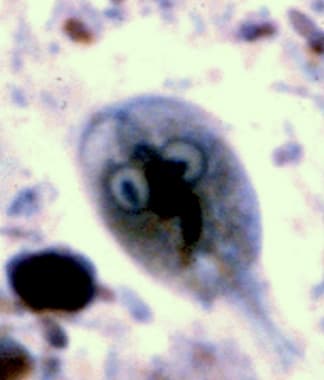The image appears to be a microscopic scan of a microorganism, characterized by a grainy, low-resolution look. Dominating the center is a large, dark purplish shape with a more solid, tadpole-like body and two round structures resembling eyes. The background is predominantly off-white with smaller, blurry specks scattered around. Various hues, including blacks, light purples, pinks, and grays, contribute to the image. The object features a distinct tail extending towards the bottom right corner, reinforcing its biological and scientific nature.